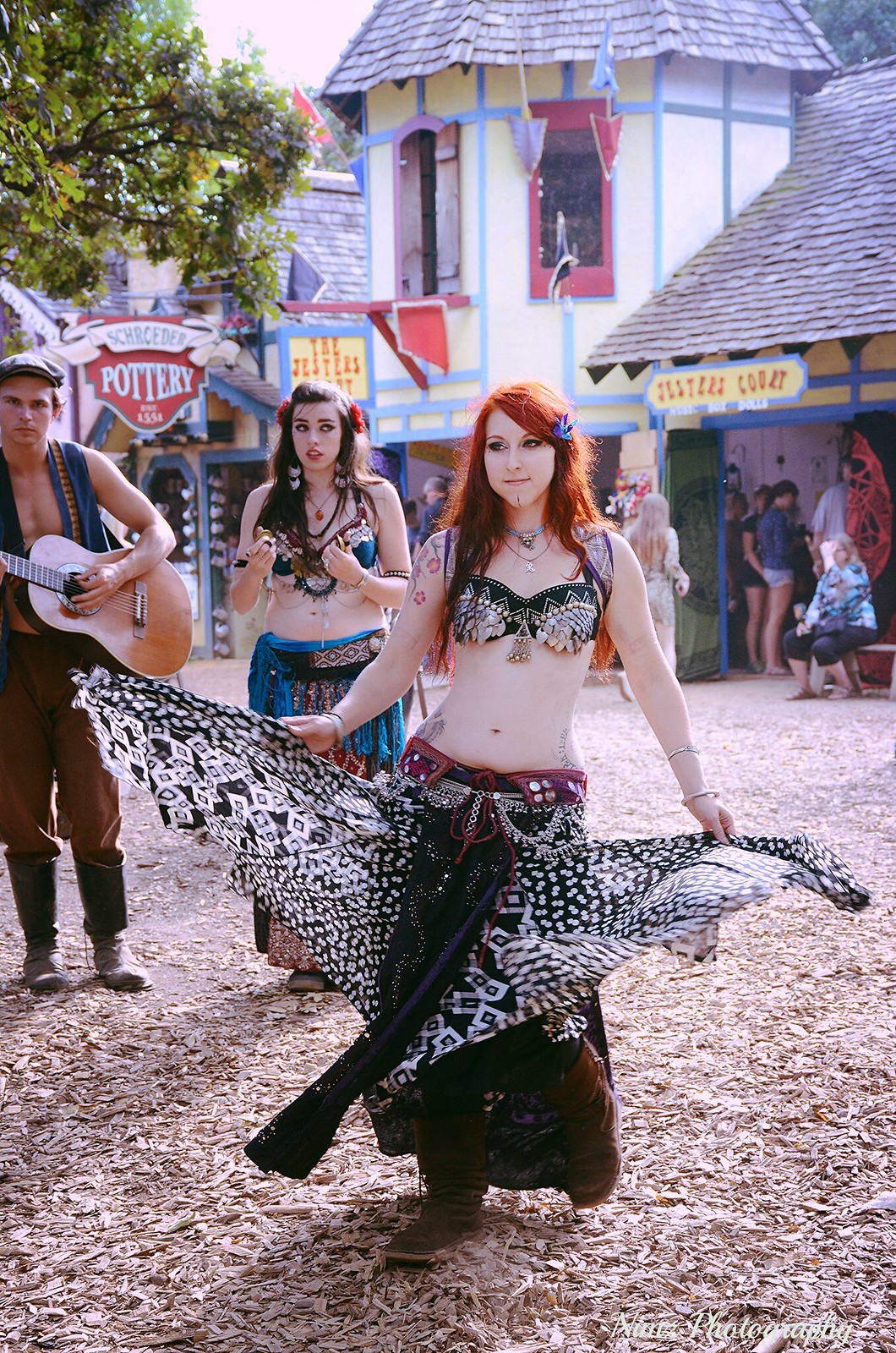This photograph captures an animated scene at what appears to be a lively medieval-themed fair or amusement park. At the center of the image, a woman with pale skin and striking red hair is absorbed in a dynamic dance routine. She is attired in a green and white bejeweled bra top, paired with dark brown to black pants adorned with frills. These frills are black and white and she’s twirling them around with her outstretched hands. She also wears brown boots and layered necklaces, and she looks off to her left as she performs.

Behind her stands another woman who also features fair skin and dark hair. She mirrors the main performer's attire but in a different color scheme, wearing a blue top and pants, accessorized with a flowing cloth. Both women give the impression of exotic belly dancers with their elaborate costumes and fluid movements.

To the left, partially cropped, is a male performer clad in a sleeveless dark blue jacket, revealing his chest, and blue hat that reflects the sunlight. He sports brown pants and black boots, and he is playing a brown acoustic guitar, seemingly in tune with the dancers. This eclectic attire and the spirited playing of the guitar suggest a festive atmosphere.

The backdrop features an old-timey two-story building with a tower-like structure. The building has a yellow façade with light blue trim and a brown tiled roof. Below the roof, there's a sign with colorful orange letters on a blue background, possibly indicating a shop or attraction. Dotted throughout the scene are people milling about, suggesting the presence of shops and restaurants, indicated by signs such as "Schroeder Pottery" and "The Jester." Green tree branches frame the left side of the image, while the ground is covered with hay or wood chips, further enhancing the rustic, medieval fair vibe.